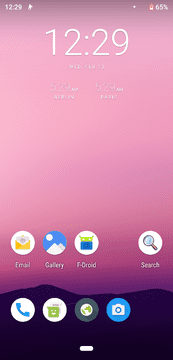This image showcases a phone's home screen set against a stunning gradient background that transitions from pink at the top to purple at the bottom, with a dark purple mountain silhouetted in the foreground. 

At the very top left, the time is displayed in white digits as "12:29" with a white app logo positioned to its right. On the top right corner, a vertical battery icon outlined in red indicates the battery level at 65% with a white fill. Centralized at the top of the screen, the time "12:29" is reiterated in white text, accompanied by the date "Saturday, February 13th" just below it. Further down, with aligned text, the current time is shown for Berlin and Paris as "5:29 AM."

Moving to the bottom, a series of app badges are neatly arranged. From left to right, there is:
1. A yellow envelope on a white circle background labeled "Email."
2. A blue circle featuring white stylized mountains and a moon, labeled "Gallery."
3. A white circle with the Android cartoon's green head, labeled "F-Droid."
4. Following a small gap, a white circle with a magnifying glass labeled "Search."

At the very bottom, four more icons are displayed:
1. A white circle with a blue phone icon.
2. A green box with a white smiley face on a white background.
3. A dark green to gray background with a greenish globe icon.
4. A blue circle with a white camera icon.

Finally, resting at the very bottom is a white pill-shaped navigation bar, completing the vibrant and visually appealing interface of the phone's home screen.